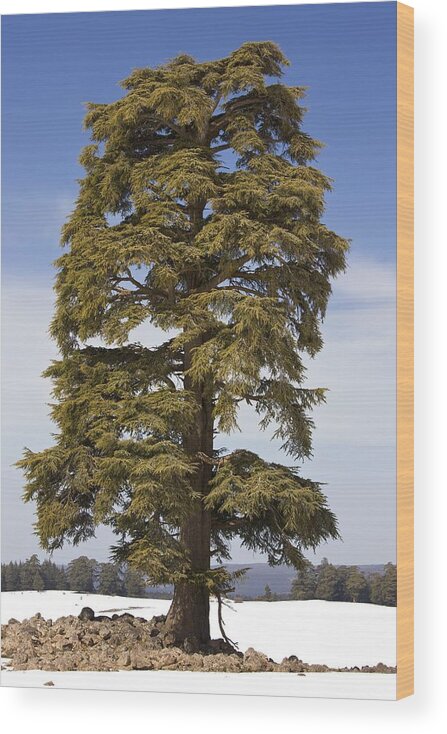The image captures a tall evergreen tree, likely a conifer, standing majestically in the center of a snowy landscape. The tree, with its vibrant forest green pine needles, bushy branches, and straight brown trunk, extends from the bottom to the top of the frame. Surrounding the tree's base are clusters of gray rocks and boulders, free from snow. In the background, a snowy field stretches out, dotted with other smaller trees, and a stunning mountain range is visible in the distance. The sky above features a gradient of wispy white clouds at the lower portion and a clear blue expanse at the top. The scene’s natural colors include shades of blue, white, green, and brown, creating a vivid and serene winter landscape. This picturesque setting, reminiscent of either a realistic painting or a high-quality photograph, places the tall tree as the focal point of the daytime outdoor scene.